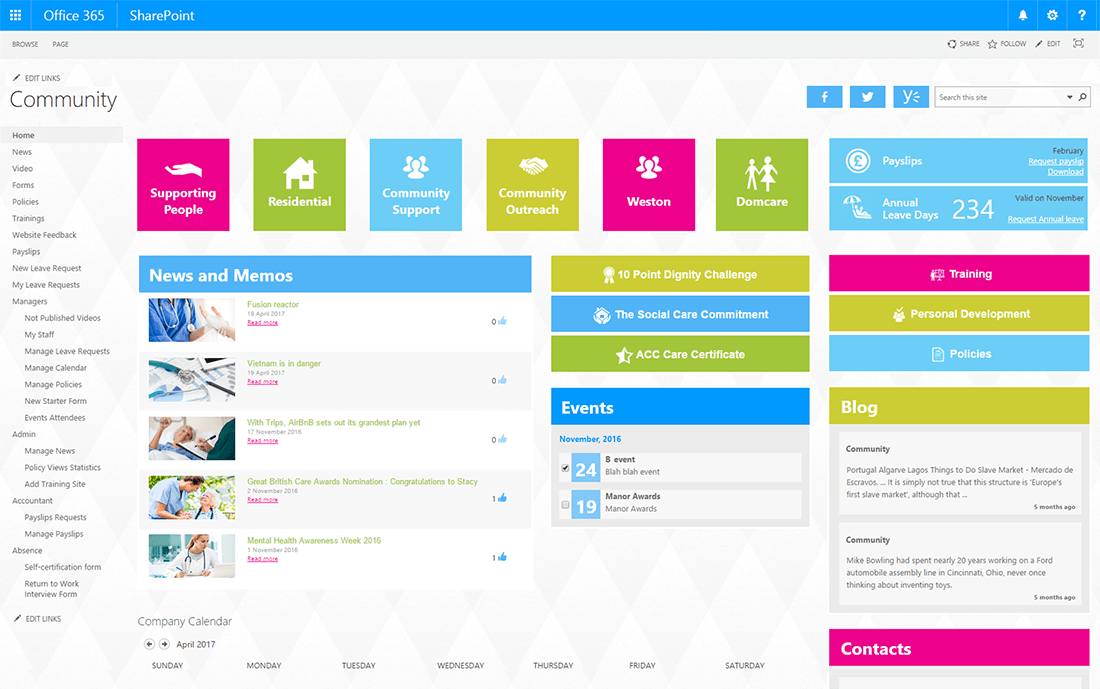This image features a white background with a structured layout. At the top, a blue banner with white text displays "Office 365 SharePoint." Below this is a gray banner with black text, listing options: "Browse," "Page," "Share," "Follow," and "Edit."

On the left side, large lettering spells out "Community," under which a vertical menu includes: "Home," "News," "Video," "Forms," "Policies," "Trainings," "Website Feedback," "Payslips," "New Leave Requests," "My Leave Requests," "Managers," and "Admin."

The central section consists of six colored boxes, each containing different text. From left to right, they are:
- Pink box: "Supporting People"
- Green box: "Residential"
- Blue box: "Community Support"
- Gold box: "Community Outreach"
- Pink box: "Westin"
- Green box: "Dom Care"

Below these boxes, there's a section titled "News and Memos," featuring headlines in green text, such as "Fusion Reactor," "Vietnam in Danger," "With Trips," "Airbnb Sets Out It's Grandest Plan Yet," among several others.

At the bottom center are rectangular buttons labeled "Ten Point Daily Challenge," "The Social Care Commitment," "ACC Care Certificate," and "Events."

On the right side, a column of buttons offers quick access to key features: "Payslips," "Annual Leave Days" (showing a count of 234), "Training," "Personal Development Policies," and "Blog."